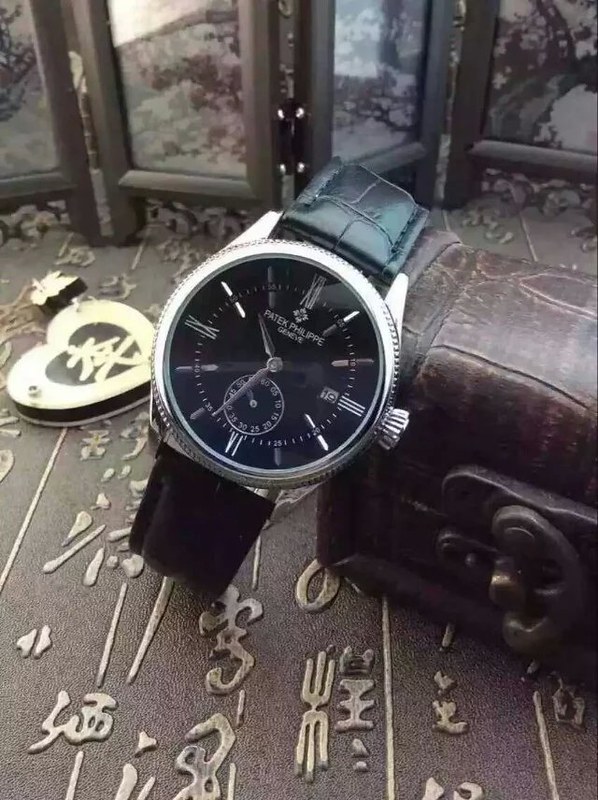The image showcases a distinguished Patek Philippe watch prominently displayed on a jewelry stand that embodies traditional Japanese aesthetics. The watch serves as the focal point, leaning gracefully against a brown leather chest that harmonizes with the background, evoking a sense of understated elegance. The background features a brown countertop, resplendently adorned with intricate gold Japanese symbols that form an elegant pattern, injecting a touch of cultural richness into the scene.

In the distance, a folding glass mirror is partially visible, poised for use to help its owner admire and adjust their jewelry with ease. To the left of the watch, adding to the traditional decor, stands a small heart-shaped ornament inscribed with a classic Japanese symbol.

The Patek Philippe itself is a picture of timeless craftsmanship, boasting a sleek black watch face paired with a slender silver bezel. The band, featuring a textured, crackly leather finish, adds a touch of sophistication, completing this harmonious blend of luxury and tradition. The meticulously arranged elements collectively evoke a serene, refined atmosphere, reflective of both Japanese culture and the exquisite taste of the watch's owner.